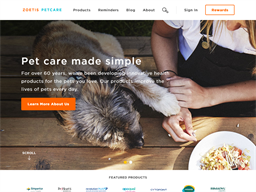In the top left corner of the image, there's an orange and blue name that is unfortunately too blurry to read. Beneath it, there's a menu listing several items, also blurred and unreadable. An orange button labeled "Pet Care Made Simple" stands out amid the blurred text. Below this button, additional unreadable text is present. The image features a brown and white dog with a black nose, alongside a person dressed in a white shirt and black overalls, sitting on a wooden patio or deck. The person is wearing a ring on one of their fingers. Nearby, a bowl of food is placed, suggesting a moment of pet care or feeding. At the bottom of the image, a series of brand logos or icons appear, but they too are too blurry to identify.